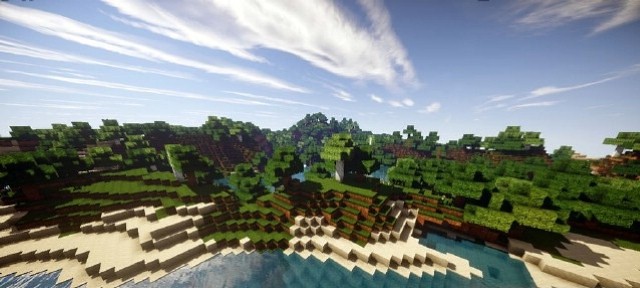This image appears to be a panoramic view inspired by the popular video game Minecraft. The scene is characterized by its blocky aesthetic, typical of Minecraft, but with a twist. The sky features a vibrant blue backdrop interspersed with clouds that are more intricately detailed than the standard Minecraft clouds, suggesting they might be superimposed to enhance the visual appeal. 

The landscape below showcases a lush, green terrain. Prominent in the scene are brown cliffs topped with verdant grass, creating a striking contrast with the land below. While it's challenging to ascertain from this image, it seems that there might be some structures built with green blocks nestled within the landscape.

Additionally, there is a noticeable body of blue water, framed by sandy edges, adding a natural and serene element to the otherwise structured environment. The overall composition of the image captures a harmonious blend of natural and constructed beauty, characteristic of a typical Minecraft landscape but with enhanced visual details.